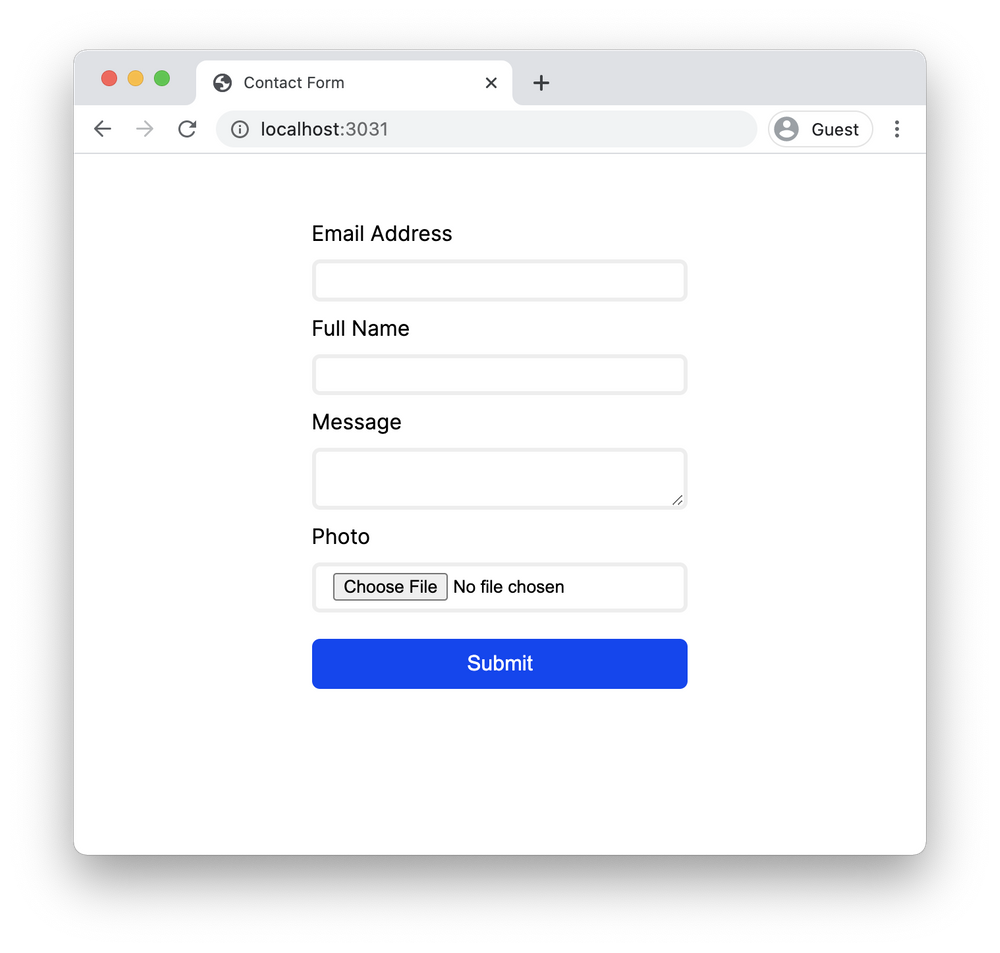The image displays a web browser, which appears to be either Safari or Chrome, being used on a MacBook or some type of Mac desktop. The top area features a light gray header typical of macOS applications. Towards the left side of this header, there are the traditional window control circles in red, yellow, and green. 

Just to the right of these circles, the active tab, labeled with a gray globe icon and "Contact Form" in dark gray text, is visible. Next to the tab is a white bar containing navigation controls: a gray left arrow symbolizing the back button and a right arrow for the forward button, which is disabled, indicating this is the most recent page. There is also a refresh symbol.

Further along this bar, there is a long, oval-shaped, light gray area with a gray-bordered circle containing a lowercase 'i' for additional information. The address bar next to it displays "localhost:3031" in black text with the colon and "3031" in gray.

On the right side of the bar, there's a light gray bordered oval featuring a gray and white silhouette of a user with the label "Guest" in black text. To the right of this, three vertical dots imply an expandable sub-menu.

The primary focus of the page is a contact form with several fields. The first field, labeled "Email Address" in large black text, has a rectangular box with a light gray border below it. Following this, the "Full Name" field is presented in the same style. Lastly, the "Message" field, also rectangular with a light gray border, is noticeably larger, approximately double the height of the previous fields. In the right corner of the message box, there are two black lines, with the second line being significantly shorter than the first.

Overall, the layout is clean and functional, clearly designed for user input through a basic contact form.